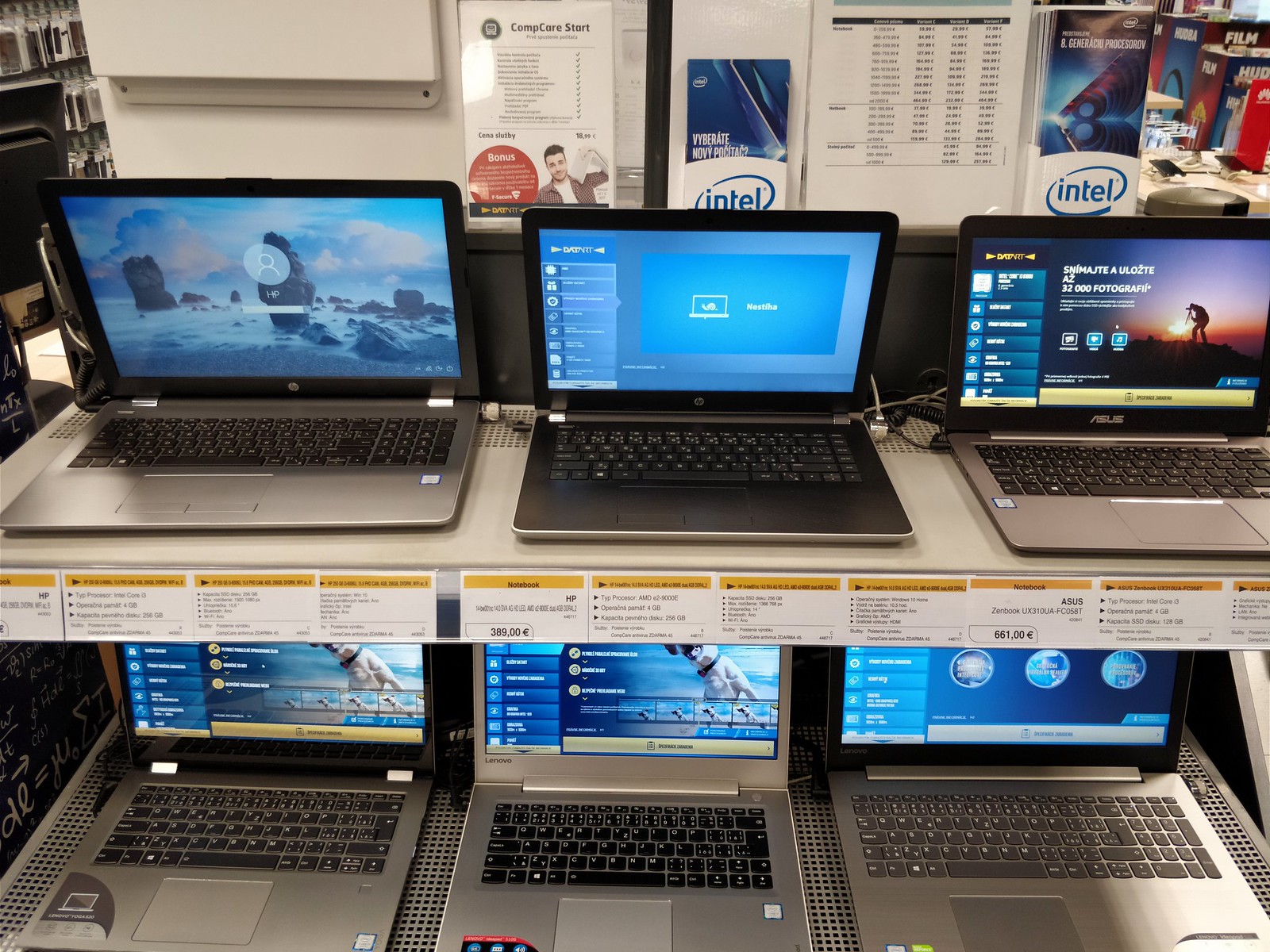This photograph captures a retail setting within a laptop section, featuring two white metal shelves in front of a wall adorned with Intel flyers, price sheets, and repair prices. The top shelf displays three mid-2010s laptops: an HP laptop on the left, a smaller HP in the center, and an Asus laptop on the right, all equipped with what appears to be Windows 10. The bottom shelf also holds three laptops, identified as possibly Lenovo models, with detailed specification sheets and price information positioned beneath them. The display provides a clear and organized view of the laptops, highlighting their features and pricing to potential buyers.